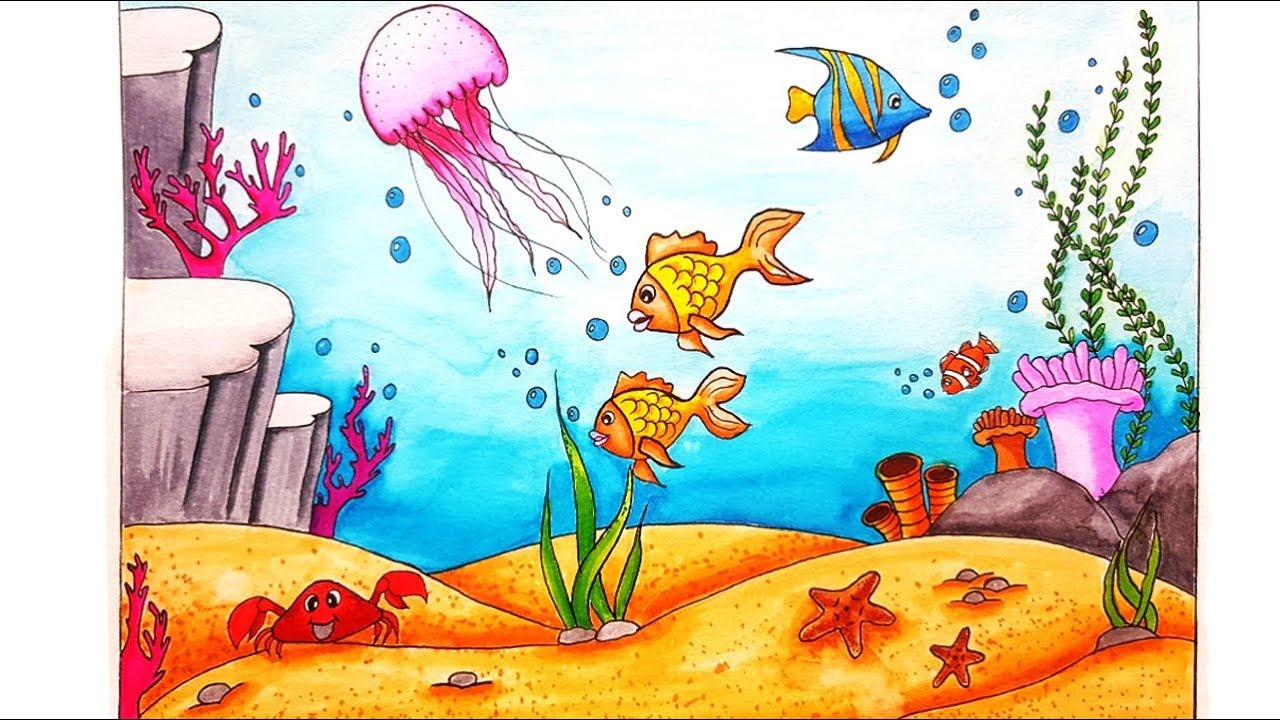This artwork captures a vibrant underwater scene, blending drawing and watercolor techniques to create a lively and colorful depiction. The sandy bottom is a warm yellow-orange, dotted with two starfish, one larger than the other, and a small red crab situated in the bottom left corner. Various marine plants are scattered throughout, including green algae, orange and pink marine plant life, and pink sea corals. To the left are rocky outcroppings with flat tops in light gray.

A pink jellyfish with long tendrils floats in the upper left, contrasting with the background, which fades from bright blue at the top to white and then darker blue towards the sandy bottom. Toward the upper right, a blue and yellow striped saltwater angelfish swims, while in the center, two goldfish of differing sizes glide side by side. In the background, an orange and white clownfish peeks out. Dark blue bubbles rise around the fish, enhancing the dynamic sense of underwater movement. The style of this art piece is cartoonish yet retains elements of realism through detailed shading and vibrant, bold colors.